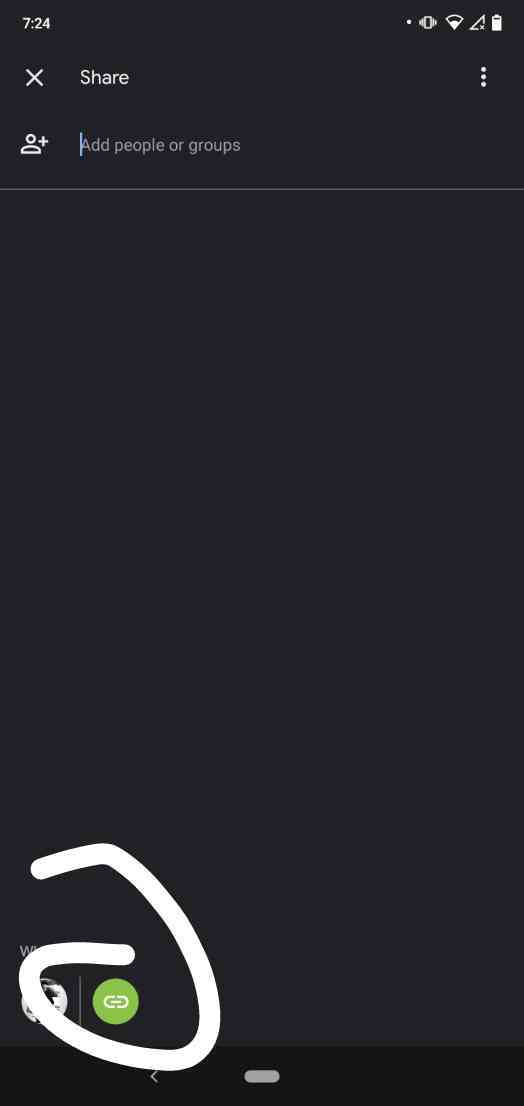This vertically rectangular image features a black background and appears to be a screenshot from a cell phone. At the top-left corner, the time is displayed as 7:24. The upper-right corner contains multiple icons, including those for phone on vibrate, Wi-Fi, signal strength, and battery level. Directly beneath the time, a large "X" is visible, followed by the word "Share" toward the center. Adjacent to "Share" on the far right are three vertical dots indicating a menu.

Below these elements, on the left side, there is an icon resembling people with a plus sign beside it, and a text field labeled "Add people or groups." The main area beneath this field is entirely empty. At the very bottom of the frame, on the left side, there are two side-by-side icons. The left icon is obscured, partially covered by a manually drawn large white circle that encircles a green link icon next to it.